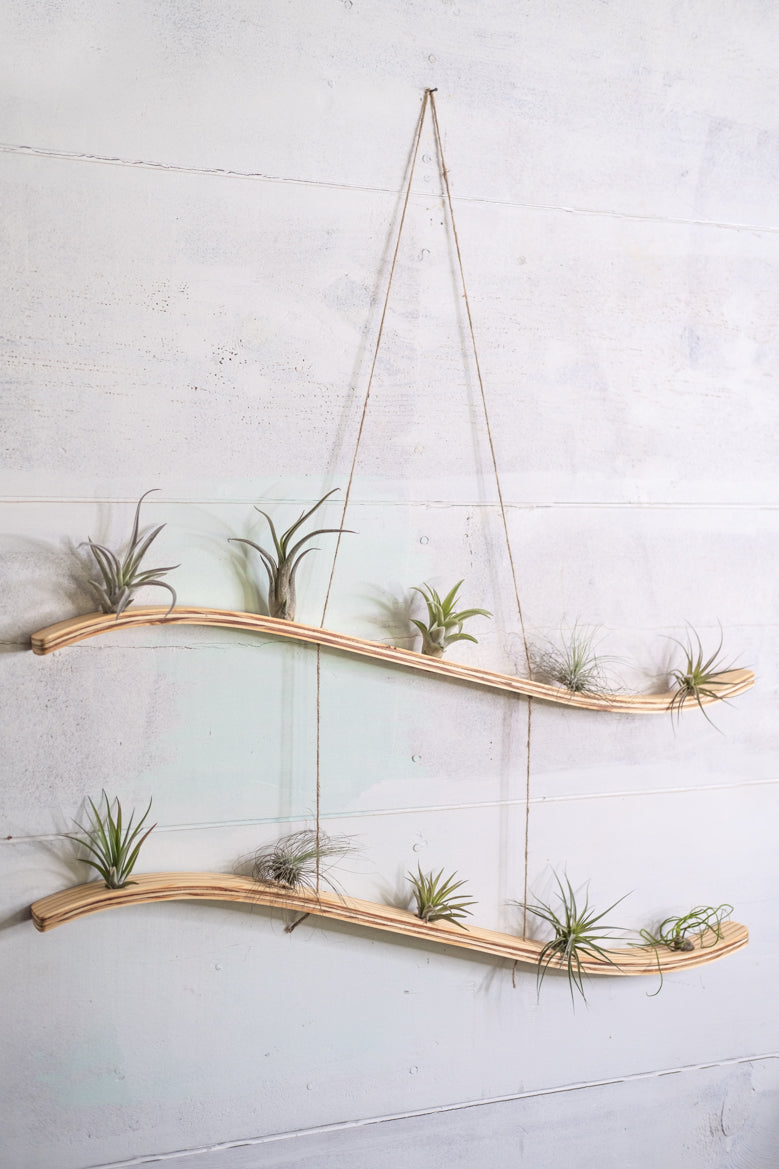This photograph showcases an artistic and functional wall-mounted plant holder. The structure comprises two elegantly curved wooden shelves, described as long slats of wood. These shelves are situated on a flat, white plaster wall and are held together by a piece of twine that forms a V-shape, extending upward to hang on a nail.

The curved design of the wood starts with an upward slope on the left, dips gently in the middle, and curves back up on the right, creating an elegant wave-like pattern. Each of these shelves contains five small holes, housing green air plants that do not require regular watering, hence no water dishes are attached. The small, cactus-like plants appear healthy and vibrant, with one plant being notably wispier than the others. The design makes it seem as though the plants are growing directly out of the wood, adding to the uniqueness of this wall art. 

The combination of natural elements with the minimalist aesthetic of the curved wood and green plants makes this wall shelf not only a practical plant holder but also a striking piece of decor.